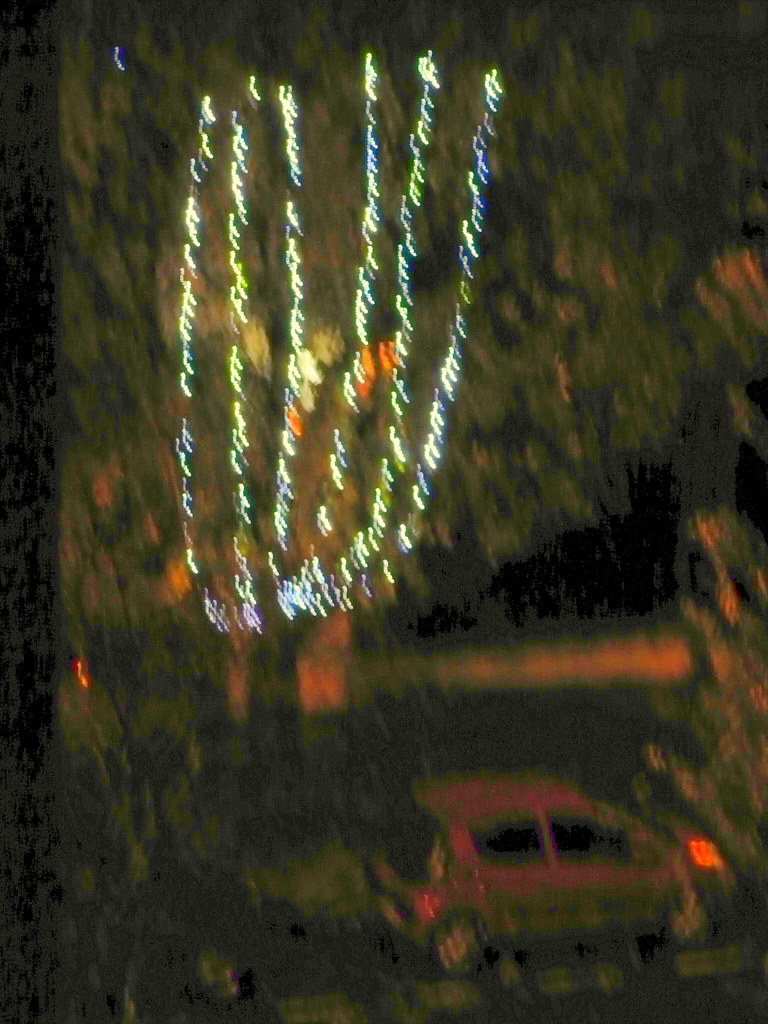A nighttime photograph capturing a festive scene, likely featuring Christmas lights, adorns a large deciduous tree. The display includes approximately six colorful strands of lights—red, blue, yellow, and purple—spiraling upwards from the trunk, creating a vibrant spectacle reminiscent of menorah prongs but without representing the menorah. A red compact car stands parked at street level, slightly offset to the right. Dense foliage partially obscures the view on the left side of the image, adding a layer of depth to the composition. The dark atmosphere accentuates the luminous decorations, emphasizing the celebratory ambiance.